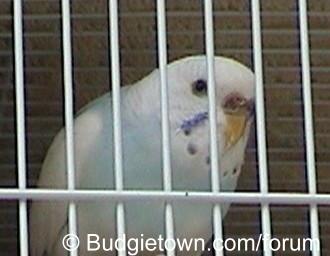This colored photo captures a close-up of a small bird inside a white cage with a vertical and one horizontal bar framing the bird. The bird, roughly the size of a parakeet or canary, stands out with its predominantly white feathers, accented by light blue on its chest and a few black spots around its neck. Its beak is a pale yellow, and only one eye is visible as the bird is turned to the side. The backdrop is a brick wall. At the bottom of the image, there is a watermark that reads "copyright budgetown.com/forum."